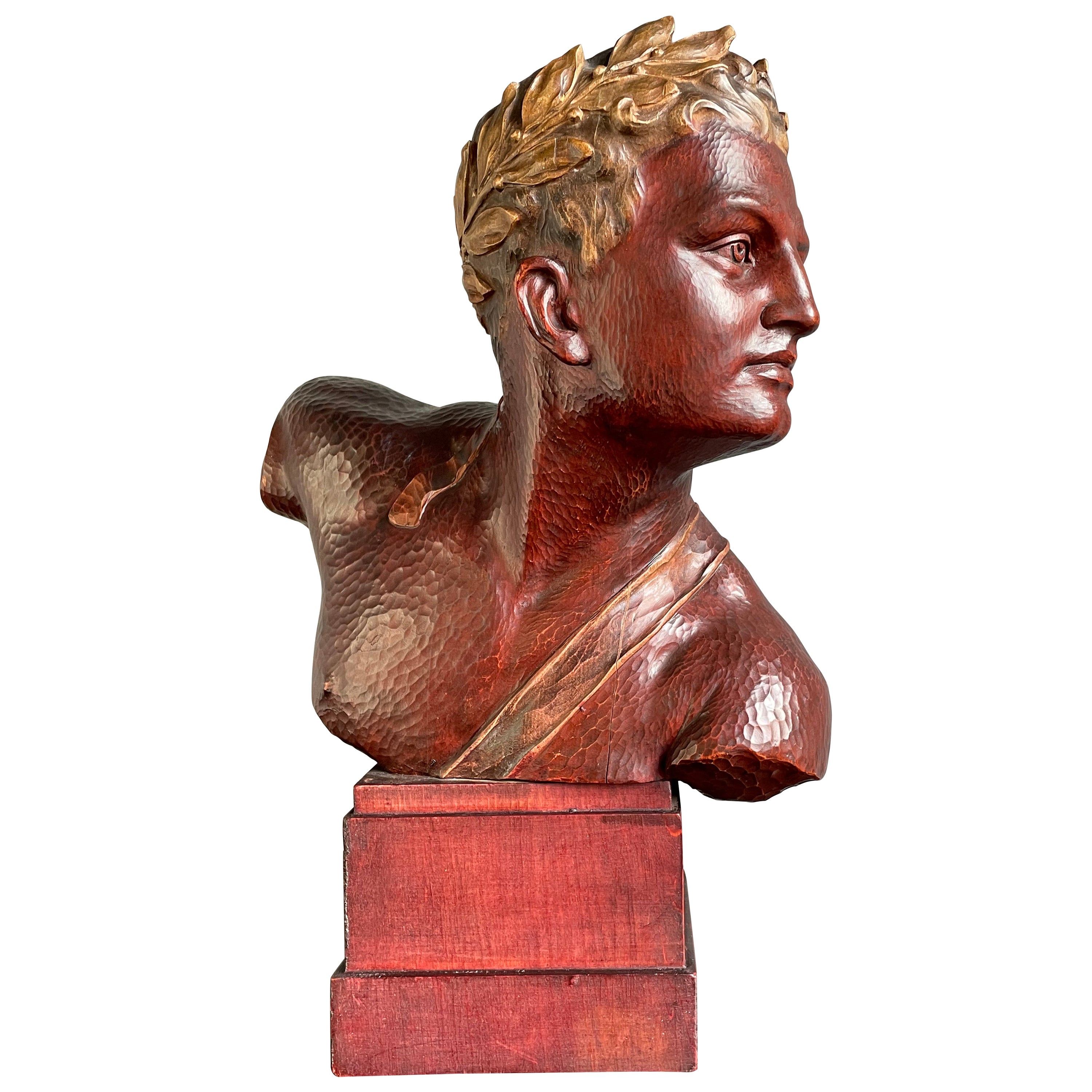The image portrays a highly detailed bust of a young person, possibly depicting a Roman or Greek figure, positioned on a reddish-brown wooden platform. The platform consists of a solid, medium-brown square base and a taller square top with a thin surface supporting the statue. The bust, which is predominantly dark brown and textured, shows the upper body with the arms appearing chopped off at the shoulders. A distinctive strap runs diagonally across the chest from the right shoulder. The figure's head, adorned with light brown, leaf-patterned hair, tilts slightly to the right, creating the impression of looking over the left shoulder. Though the material of the sculpture is unclear, it may be made of bronze or a similar metal, with the skin subtly tinted reddish. All features, including open eyes and precisely detailed facial characteristics, convey a realistic appearance, set against a plain white background.